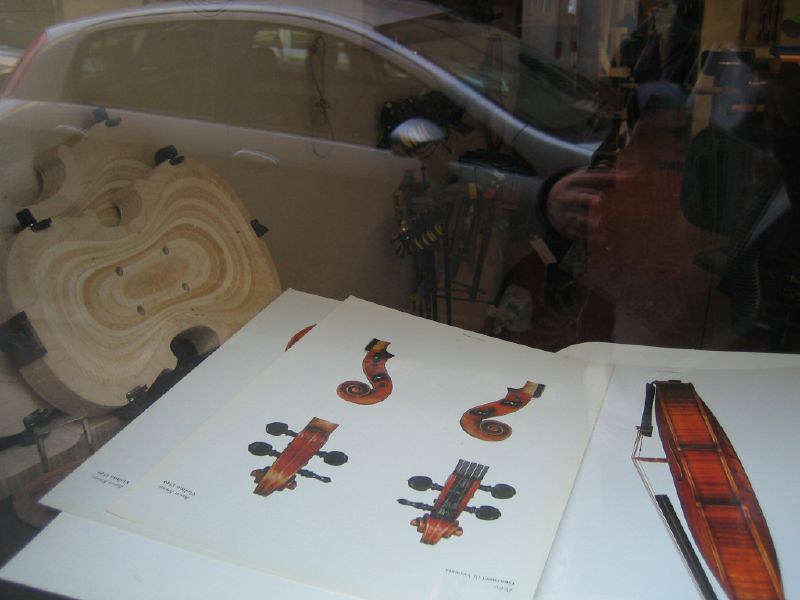The image depicts a scene from outside a violin-making workshop, as observed through a reflective window. Dominating the foreground is the glass reflection of a parked four-door coupe and a hand, possibly belonging to the person taking the photo, along with a blue baseball cap and black sunglasses. Inside the establishment, multiple sheets of paper lie on a flat surface, containing detailed sketches and drawings of various parts of a violin. On the leftmost paper, a design showcases the intricately curved handle of a violin, complete with multiple adjustment knobs on each side. Adjacent sheets feature side and profile views of a string musical instrument, potentially a violin or fiddle, highlighting the placement of the strings and the dark bases they rest on. Also visible in the workshop is a partially constructed violin body, made of light brown wood and secured with clamps, possibly mid-construction. The inner depths of the workshop, though somewhat obscured by the reflections, reveal a white wall and what appears to be a wooden decorative piece, oak-colored with visible grain and dark metal attachments, possibly another part of a stringed instrument, such as a violin or cello.